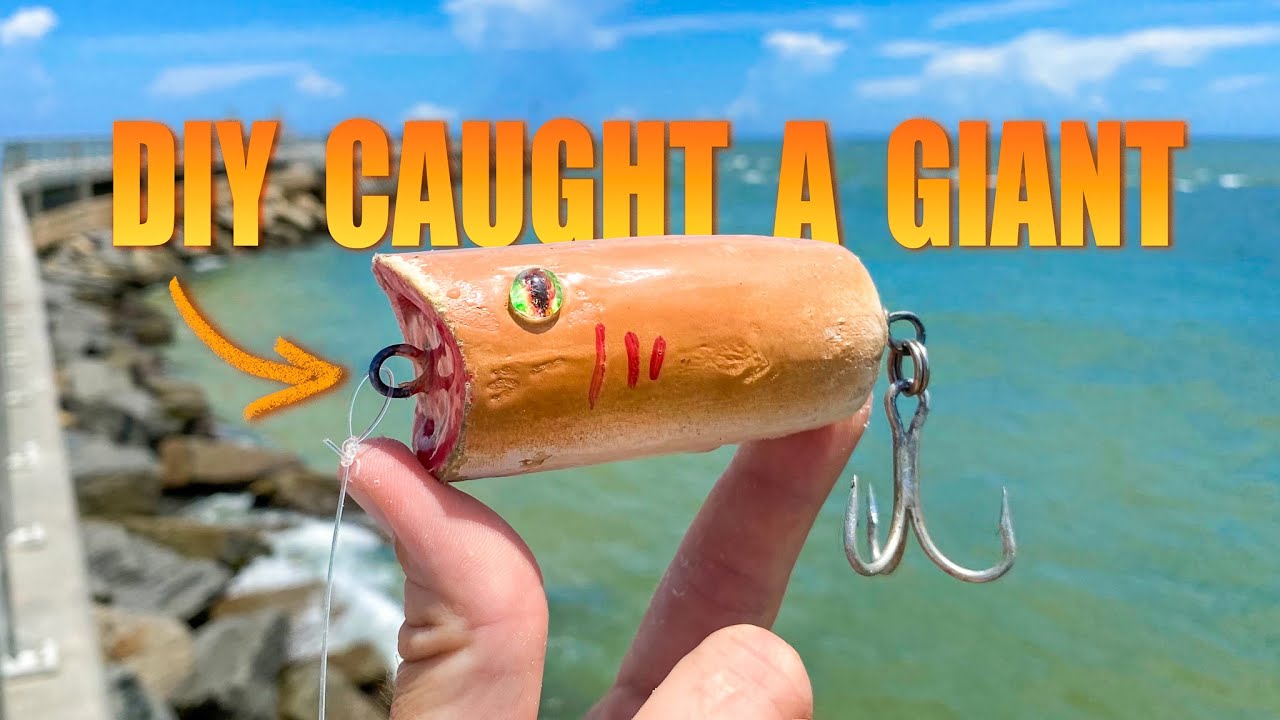The image shows a person holding up a DIY fishing lure with their left hand, pinched between their thumb and index finger. The lure resembles an orange hot dog and features a fish-like eye and red gills, with a hook area around the eyelet for attaching a string on the left side. The right side of the lure has three dangling hooks. Above the lure, in orange letters, is the text "DIY caught a giant," with an arrow pointing to the lure beneath "DIY." The background includes a greenish-blue ocean to the right, a rocky shoreline to the left, and a blue sky with wispy white clouds above the horizon. There appears to be a pier in the background and possibly a guard rail along the shore, suggesting it's along a walking path or road.